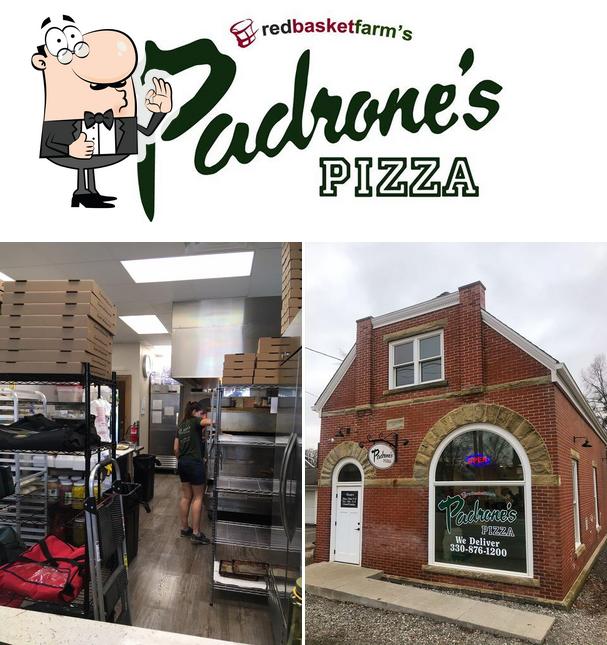The webpage features a three-panel layout with a prominently displayed top bar, followed by two side-by-side panels containing images. At the top of the webpage, the company name "Red Basket Farms" is showcased in a stylized, curved font. "Red" is in a combination of red and black, "Basket" in burgundy, and "Farms" in green. A stylized basket is positioned to the side of the company name, enhancing the branding.

Below the company name, there is a cartoon rendering of a male figure dressed in a tuxedo, complete with pointy shoes, a mustache, a bulbous nose, and googly eyes. His eyebrows are offset from his face, and he has a small amount of hair at the back of his head. The character is giving a thumbs-up with his right hand and making an okay sign with his left hand. This figure is superimposed over the logo of "Padrones Pizza." The "Padrones" text is in a brush-style font with a slight rightward slant, while "Pizza" is outlined in black capital letters with a white fill.

The left panel below shows the interior of a pizza restaurant. It includes a worker, trays, and empty pizza boxes within a partially visible workstation that features a wood-grained floor. 

The right panel depicts the exterior of a red brick building with a pitched roof on both sides, an upper window, and an arched white front door and window featuring the "Padrones Pizza" sign. The building is set on a gravel ground with a sidewalk leading out to the left, which abruptly stops without connecting to any other path. The windows and doors are elaborately framed with arched stonework. The red brick building also has two solid vertical extensions on the side that are partially visible. The sign on the building includes the contact information, "30876-1200", indicating that they offer delivery services.